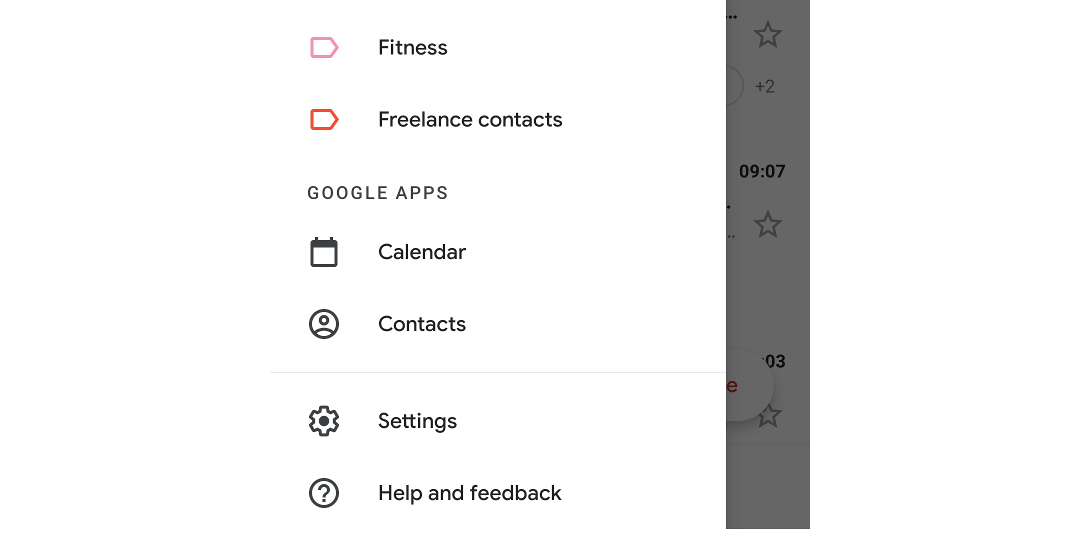This screenshot features a predominantly white background. On the left side, there is a unique pink square with a pointed middle on its right edge. Adjacent to this icon, the word "Fitness" is prominently displayed in bold black text. Below it, a similar shape appears in red, accompanied by the text "Freelance Contacts" to its right. These two sections are separated by approximately five rows of spacing.

Further down, about four lines below the previous content, the text "GOOGLE APPS" is presented in all caps and in gray. Underneath this heading, a series of icons are aligned vertically on the left, each followed by their respective names to the right: "Calendar" and "Contacts." A thin, light gray horizontal line separates these from the next set: "Settings" and "Help and Feedback."

On the right-hand side of the screen, a dark gray vertical rectangle stretches from the top to the bottom. This column is decorated with star outlines in gray. The first star appears at the top, followed by another star situated approximately four lines down, accompanied by a "plus sign two" notation. About five lines further down, a bolded timestamp "09:07" is displayed. Approximately three lines below this, another star is positioned, followed by a bolded "03" about eight lines down, with yet another star four lines beneath that.